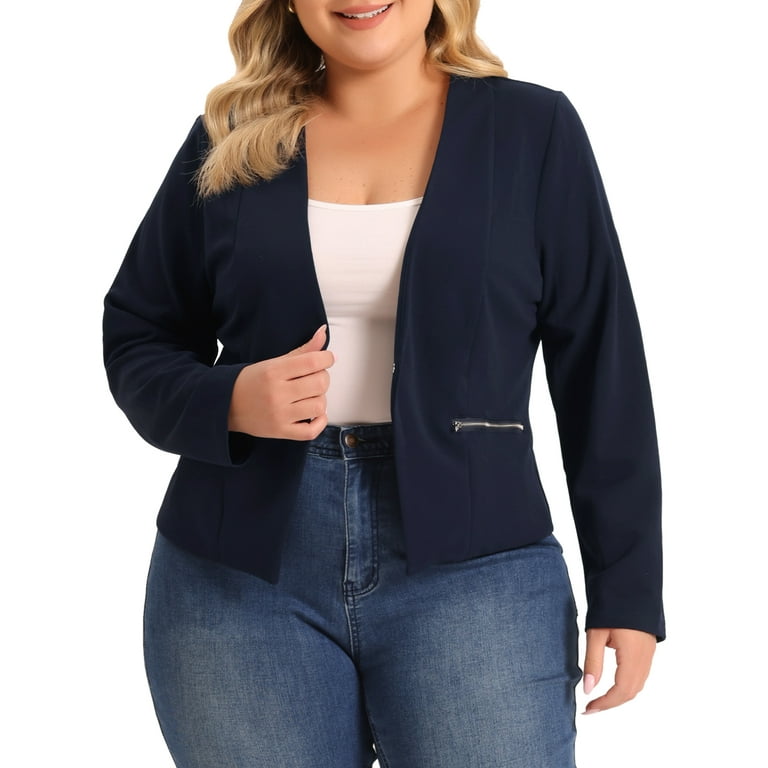The image displays the torso of a plus-sized woman with long blonde hair, smiling softly against a solid white background. Gold loop earrings adorn at least one of her ears. She is dressed in a white top, possibly a halter or tank style, tucked into snug, stonewashed blue jeans that fit her mid-thigh and lack a belt. Over the white top, she wears a dark navy blue jacket with silver zippered pockets on each side. Her right hand holds the waist of the jacket, while her left arm hangs naturally by her side. Her fingernails are painted a delicate pink, adding a touch of elegance to her casual yet stylish outfit. The significant colors in the image include shades of blue, white, the flesh tones of her skin, and the pink of her nails, making for a harmonious, appealing visual likely intended to display the outfit for commercial purposes.